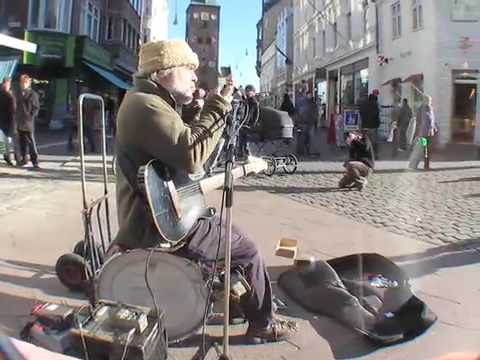This color photograph captures a close-up of a street performer, possibly a busker, seated on a street corner in a bustling city lined with high-rise buildings. The artist is dressed in vibrant, eclectic winter clothing: a yellow fluffy knit hat covering his ears, a long-sleeved olive green jacket, and purple pants paired with brown, boot-style shoes. He sits atop a large bass drum, cradling a black electric guitar in his lap, which is strapped over his shoulder. In front of him, a microphone stands ready, connected to a nearby battery-powered amplifier, indicating his setup for live performance. A black tarp and an open cloth guitar case are spread out in front of him for collecting tips from passersby. A moving dolly and various other gear items are positioned behind him. Several onlookers are gathered nearby, capturing a moment of city life centered around this colorful, musical street scene.